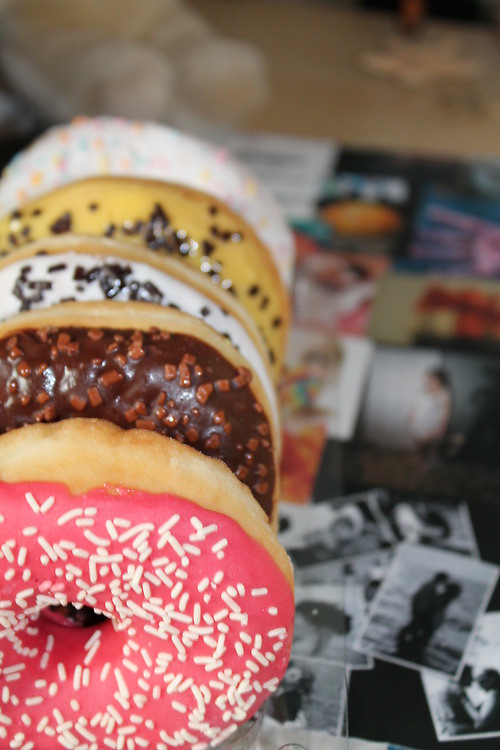This is a close-up photograph of five visually appealing doughnuts, each stacked upright in a neat row along the left side of the image. The doughnuts vary in appearance: the one in the front features white bread with a glossy pink glaze and white sprinkles. Directly behind it is a doughnut with a light bread topped with chocolate frosting and brown sprinkles, possibly mixed with chopped nuts. The third doughnut shows a light brown bread adorned with white frosting and brown chocolate sprinkles, while the fourth doughnut stands out with a yellow glaze and chocolate sprinkles. The last doughnut, furthest back, has a white glaze with colorful pastel sprinkles scattered on top.

In the blurred background, there's a table covered with an assortment of photographs, some in color and others in black and white. These images display various people and scenes, including a couple embracing on a beach, a person wearing sunglasses, and possibly a little girl with voluminous hair. Also faintly visible near the top of the background, another table appears to hold more doughnut-like desserts arranged on a tray. The overall setting is simple yet engaging, offering a tantalizing glimpse of both the vibrantly decorated doughnuts and the nostalgic photographs behind them.